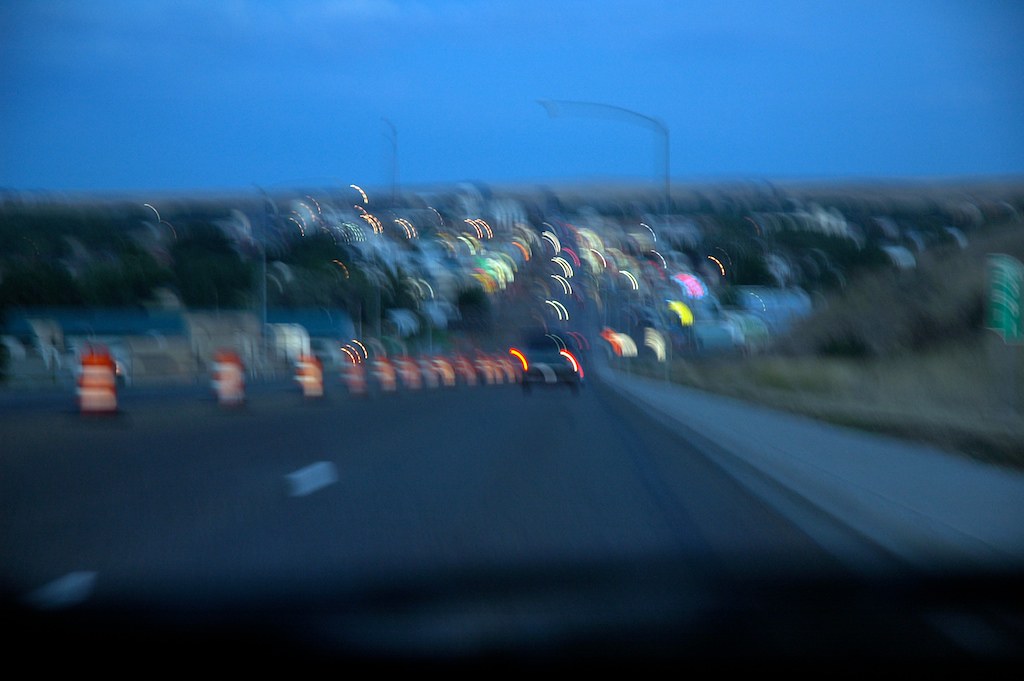A rectangular, landscape-oriented photograph captures a nocturnal street scene, though the image is notably blurry. Dominating the background is a dark gray truck, positioned ahead on the dimly lit road. On the left-hand side of the street, a series of orange construction barrels are neatly aligned, creating a sense of ongoing roadwork or diversion. The night sky above is a deep, inky blue, hinting at the late hour. In the distance, a variety of buildings form an urban silhouette, their windows and facades adorned with a spectrum of lights. These illuminations, in vibrant shades of pink, yellow, green, red, and white, create a mosaic of colors that contrast with the otherwise muted scene.